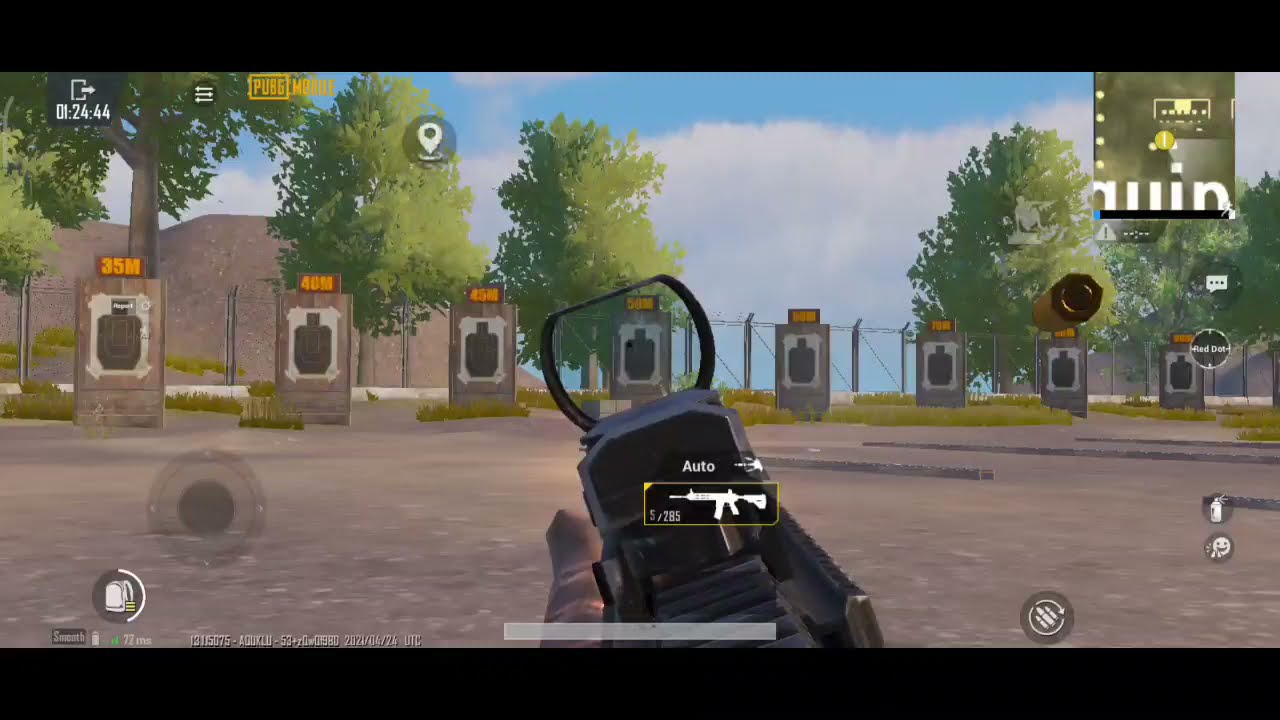This is a horizontal rectangular screenshot from the video game PUBG Mobile. The top and bottom of the image are bordered by black bars, framing the central animated scene. The scene depicts a shooting range with a concrete ground, extending into the distance. At the center bottom of the image, there's a visible portion of a vehicle, likely a motorcycle, with a small windshield and black seating.

In the middle of the screen, a black gun is aimed at a series of targets set up in a row, each affixed to vertical brown boards. These targets feature a white paper with a black shaded outline resembling a person’s torso. Above each target, yellow signs display the distance in meters: starting with 35m on the left, increasing incrementally by 5 meters, reaching up to 70m as they recede into the distance.

Additional details include a chain-link fence and trees visible behind the targets under a blue sky with white clouds. In the upper left-hand corner, a small square black box displays a timer (01:24:44) with a right arrow, along with the text "PUBG Mobile" in yellow. On the upper right-hand corner, another small square box with some white text is partially cut off from view.